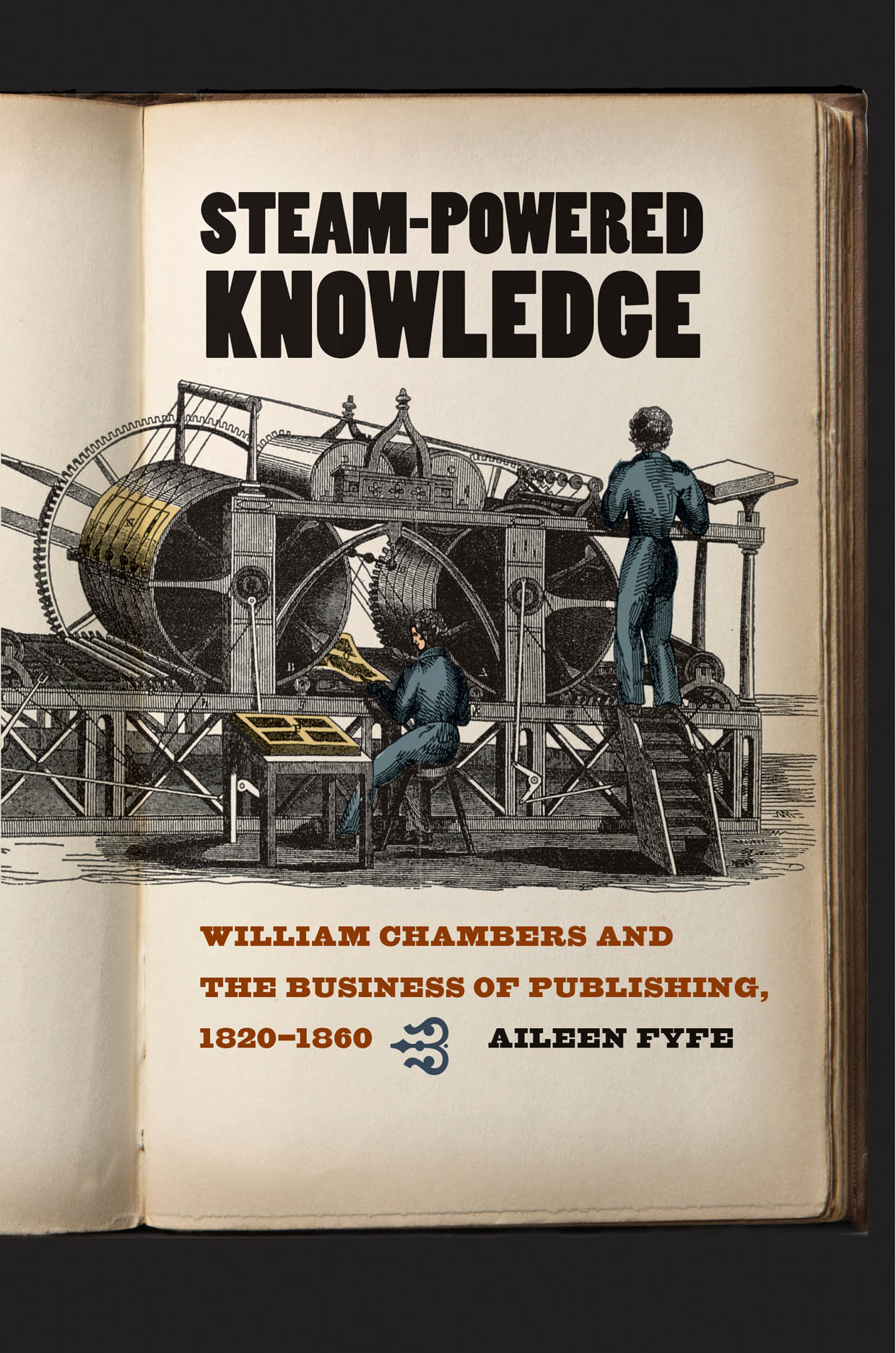The image is a detailed photograph of an old book. At the top of the book's page, bold black letters spell out "STEAM POWERED KNOWLEDGE," taking up a significant portion of space. Below this, a large, intricate image dominates a third of the page, depicting a complex steam-powered printing machine with two barrels or wheels. Two men dressed in identical uniforms are working on the machine; one is seated and tinkering, while the other is standing on a stepladder, also attending to the machine's workings. Beneath this image, red text reads "WILLIAM CHAMBERS AND THE BUSINESS OF PUBLISHING, 1820-1860," followed by a small symbol and then the name "EILEEN FYFE." The edges of the book show signs of age, adding to the sense of historical authenticity.